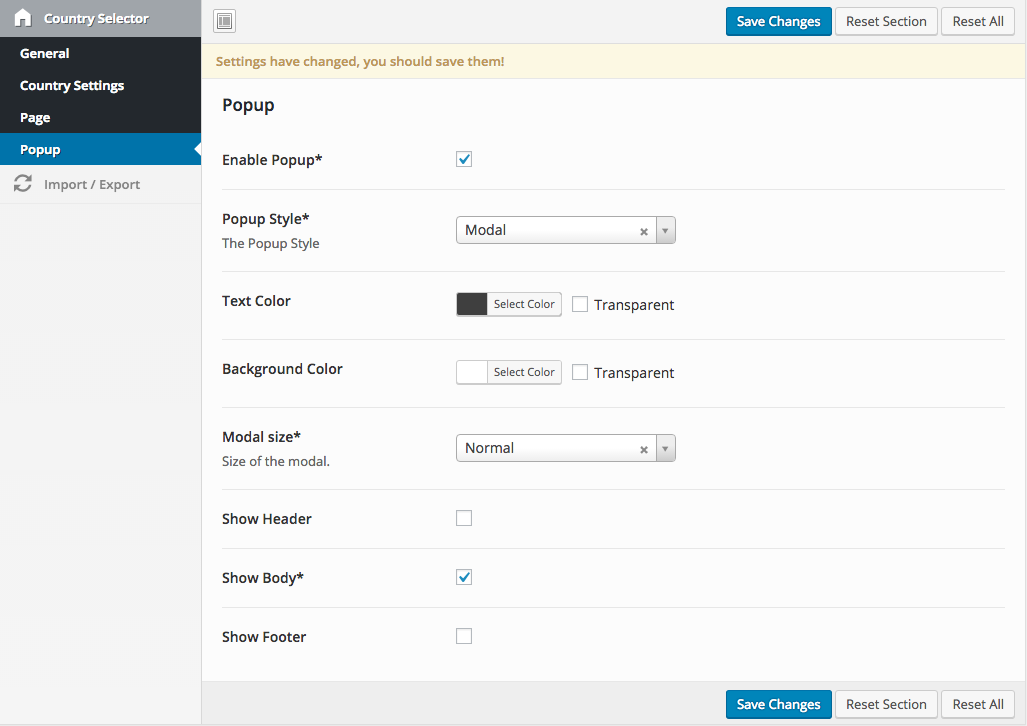In this image, we observe a user interface for configuring various settings, likely for a web application or software.

Starting from the upper left corner, there's a **Country Selector** dropdown menu, allowing users to choose their country. Below this, a series of collapsible sections are available for **General**, **Country Settings**, **Page**, and **Pop-Up** configurations.

Dominating the right side of the page, which is significantly larger, is the **Pop-Up** settings area. This includes several customization options:

- **Enable Pop-Up**: This is checked, indicating that pop-ups are activated.
- **Pop-Up Style**: Set to "Modal", which is likely designed to overlay content.
- **Text Color**: Provides selections for color and an option to make text transparent.
- **Background Color**: Default set to white with an option to make the background transparent.
- **Modal Size**: Configured to "Normal".
- **Show Header**: Unchecked, meaning the header is not displayed in the pop-up.
- **Show Body**: Checked, indicating that the body content of the pop-up is visible.
- **Show Footer**: Unchecked, meaning the footer is not displayed.

At the bottom of this section, there are three buttons: **Save Changes** (in blue), **Reset Section**, and **Reset All**. These buttons are also mirrored at the top of the page for quick access.

The overall design of the interface is clean, primarily featuring a white background with gray elements and blue accents, complemented by minimal black text and icons, which enhances readability and ease of use.

This setup appears to be a dedicated page for adjusting various settings related to country and pop-up appearances, allowing users to precisely configure their preferences.